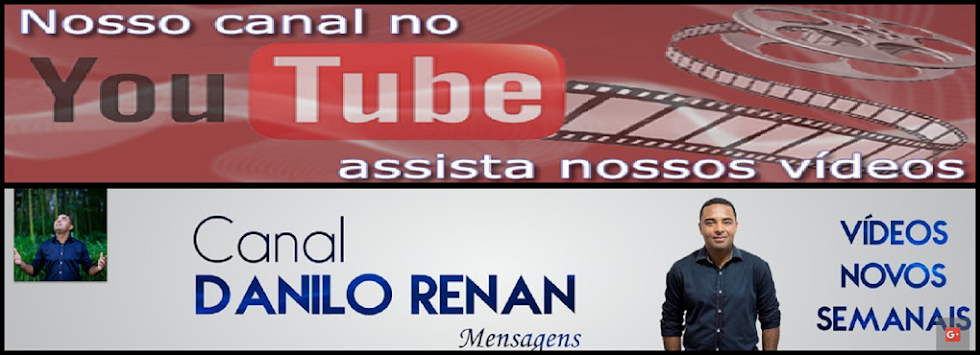The image is a wide rectangular advertisement for a YouTube channel. The upper half features a striking red background adorned with an old-style film reel spiraling across it, adding a dynamic touch. Prominently placed in the upper right of this section is the YouTube logo, with the text "NoSoCanalNo" in white letters to the upper left and "AsistaNoSosVideos" in a similar style below the logo. The lower half transitions to a light gray backdrop, where, on the right, "Videos Novos Semanas" appears in blue text over three lines. Central to this part of the image is a man with darker skin and short black hair, wearing a navy blue dress shirt, smiling directly at the camera. To the left, "Canal Danilo Renan Mensajens" is displayed in red text, accompanied by a smaller square image of the same man in the same attire, standing in a green forest with his hands open and looking upward.